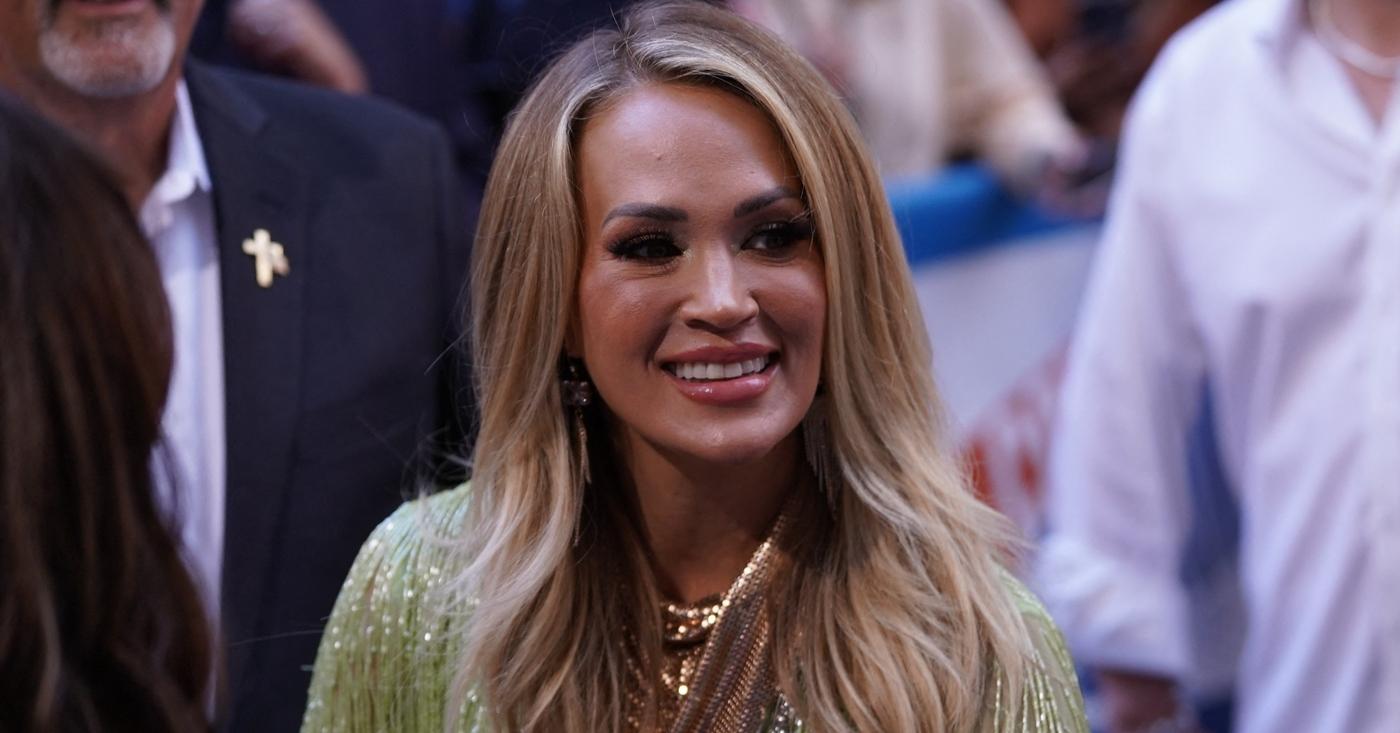The picture prominently features a woman, who is believed to be Carrie Underwood, positioned centrally in the image. She has long, light brown hair with highlights and is smiling, revealing her teeth. She is wearing a shimmery, lime green blouse with a gold collar. Her makeup includes noticeable lipstick, eye shadow, and eyebrow makeup. She accessorizes with gold-colored jewelry, including a necklace and shiny earrings. In the background, two men are visible, albeit slightly blurry: one on her right in a white button-up shirt, and another on her left wearing a suit jacket with a cross lapel pin. The image has high clarity and brightness, with ample natural light enhancing the scene.